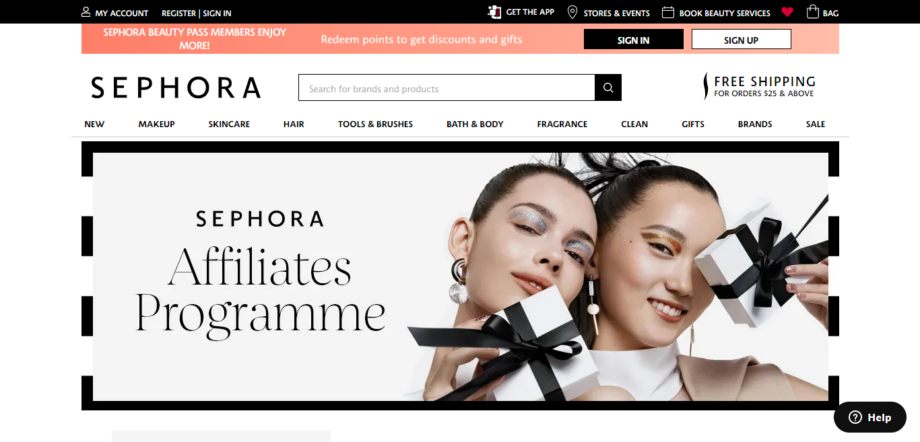The image displays a webpage with a comprehensive header and a promotional section. 

At the very top, the header includes navigational tabs. On the top left, the options are: "My Account", "Register", and "Sign In". On the top right, the available tabs are: "Get the App", "Stores & Events", "Book Beauty Services", "Bag", and a red heart icon. 

Beneath the header is a text that reads, "Sephora Beauty Pass members enjoy more redeem points, so get discounted gifts". On the right side of this text, there are two buttons: a black "Sign In" button and a white "Sign Up" button. The background for this section is pink.

The main page below has a white background. On the left side, the word "Sephora" is prominently displayed. There is a search box prompting users to "Search for brands and products". Below this, the text "Free Shipping" is visible, with additional text on the right side stating, "Free shipping for orders $25 and above".

The navigation tabs start from left to right and include: "New", "Makeup", "Skincare", "Hair", "Tools & Brushes", "Bath & Body", "Fragrance", "Clean", "Gifts", "Brands", and "Saves".

At the center of the page is a promotional section featuring the text, "Sephora Affiliates Program". Two women are shown holding white present boxes wrapped with black ribbons. Both women are wearing makeup and are set against a light gray background with a black outline at the bottom of the image. 

Additionally, there is a blue "Help" button located in the bottom left corner of the webpage.